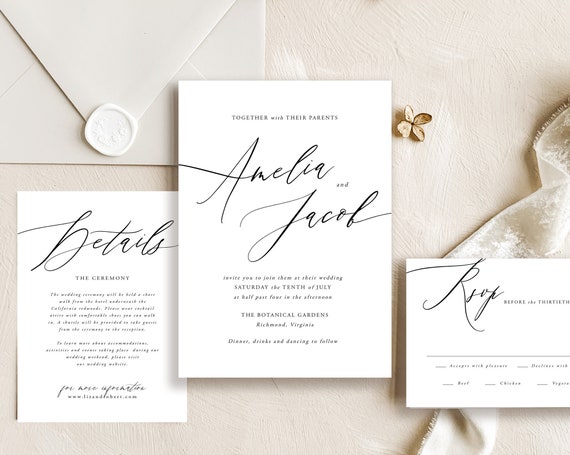The image displays a set of three wedding invitations arranged on a light brown or ivory white background. In the top left corner, a white envelope with a wax seal and a delicate marking complements the elegant theme. The invitation on the left is vertically oriented, featuring bold script at the top that appears to read "Details." It includes a few smaller paragraphs below, adding to its intricate design.

At the center, the largest invitation showcases the names "Amelia and Jacob" in an elegant black script font. Further details such as "Together with their parents," the wedding date "Saturday, the 10th of July," and the venue "Botanical Gardens in Richmond, Virginia" are presented in smaller fonts, creating an inviting and formal appearance.

To the right, a smaller, business card-shaped invitation serves as an RSVP card. It instructs guests to "RSVP before 13th" with a blank line provided for responses. The invitation layout includes a small four-petaled gold flower near the central card, alongside a curling white floral ribbon, adding a decorative flair to the overall arrangement.